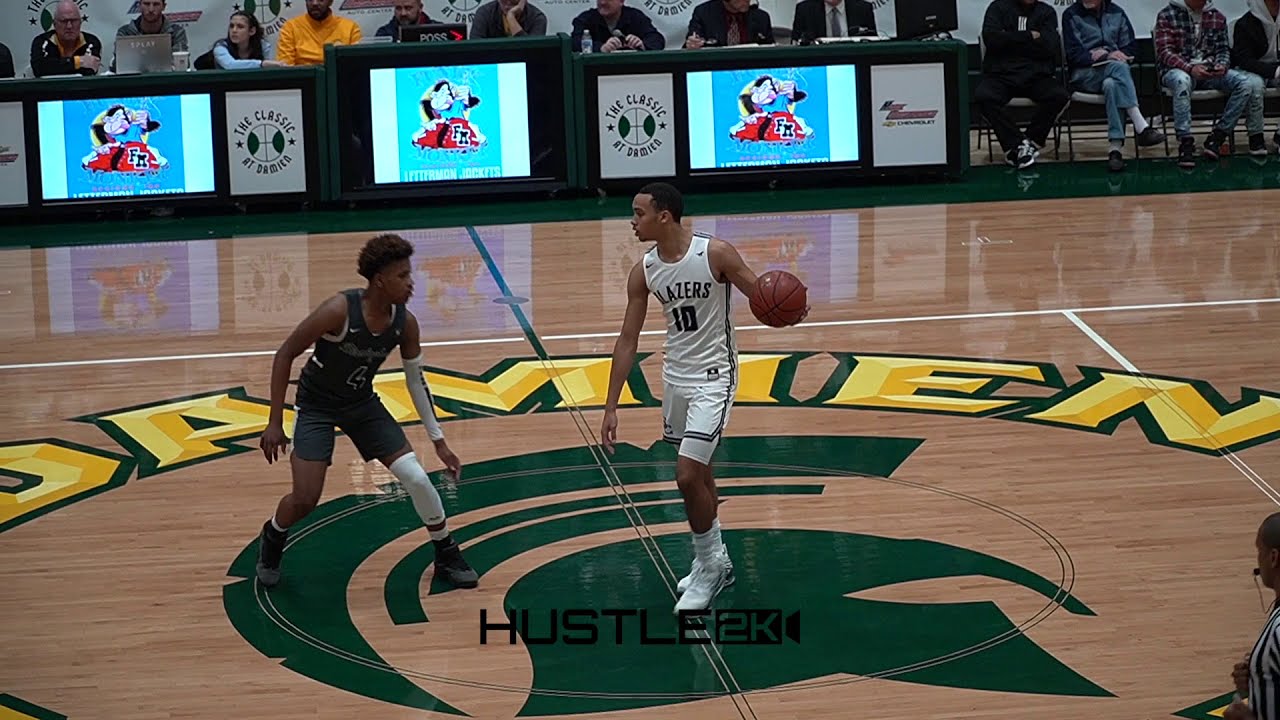This image captures a dynamic moment from a college basketball game featuring the Blazers facing off against Michigan State at Michigan State's stadium. The court prominently displays the Spartan logo in green at center court. The player on the right, in a white uniform with green trim and the number 10, is dribbling the basketball. Clearly visible is the Nike logo on his attire. He represents the Blazers, as indicated by the writing on his shirt and shorts. On the left, his opponent in a green uniform bearing the number 4 watches closely, ready to defend. In the bottom right corner, a referee with a whistle in his mouth is seen overseeing the play. In the background, spectators are seated, with some positioned behind the scorer’s table, which displays digital advertisements, including messages like "The Classic" and "Hustle 2K." The court's green borders and yellow lettering contribute to the vibrant atmosphere of this intense game moment.